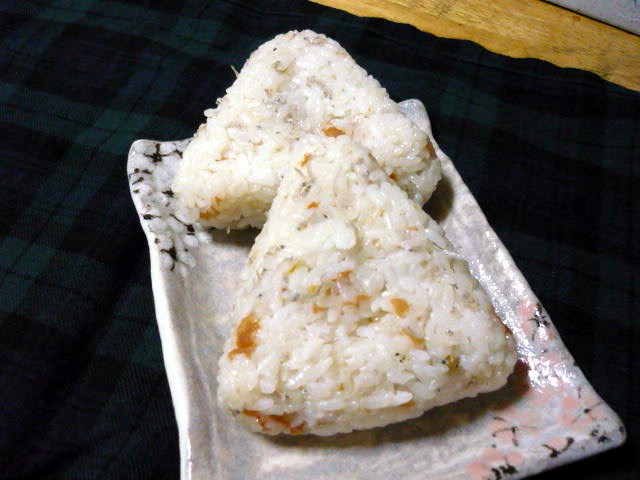This is a color photograph of two triangular cakes that resemble onigiri, presenting a unique fusion of textures. The cakes seem to be baked and then dipped or rolled in rice, revealing a hint of pastry underneath. These delightful creations rest on a rectangular, ceramic plate with a distinctly Japanese aesthetic. The plate, light gray with an opalescent sheen, features delicate cherry blossom designs—white flowers with black centers in the upper left corner, and pink blossoms adorning the right edge. The plate sits at an angle, spanning from the bottom right to the upper left of the frame. The background remains predominantly black, save for a portion of light wood that cuts diagonally across the upper right-hand corner, accompanied by a small patch of gray. The photograph, likely a casual snapshot, captures the serene and delicate arrangement with no text present.